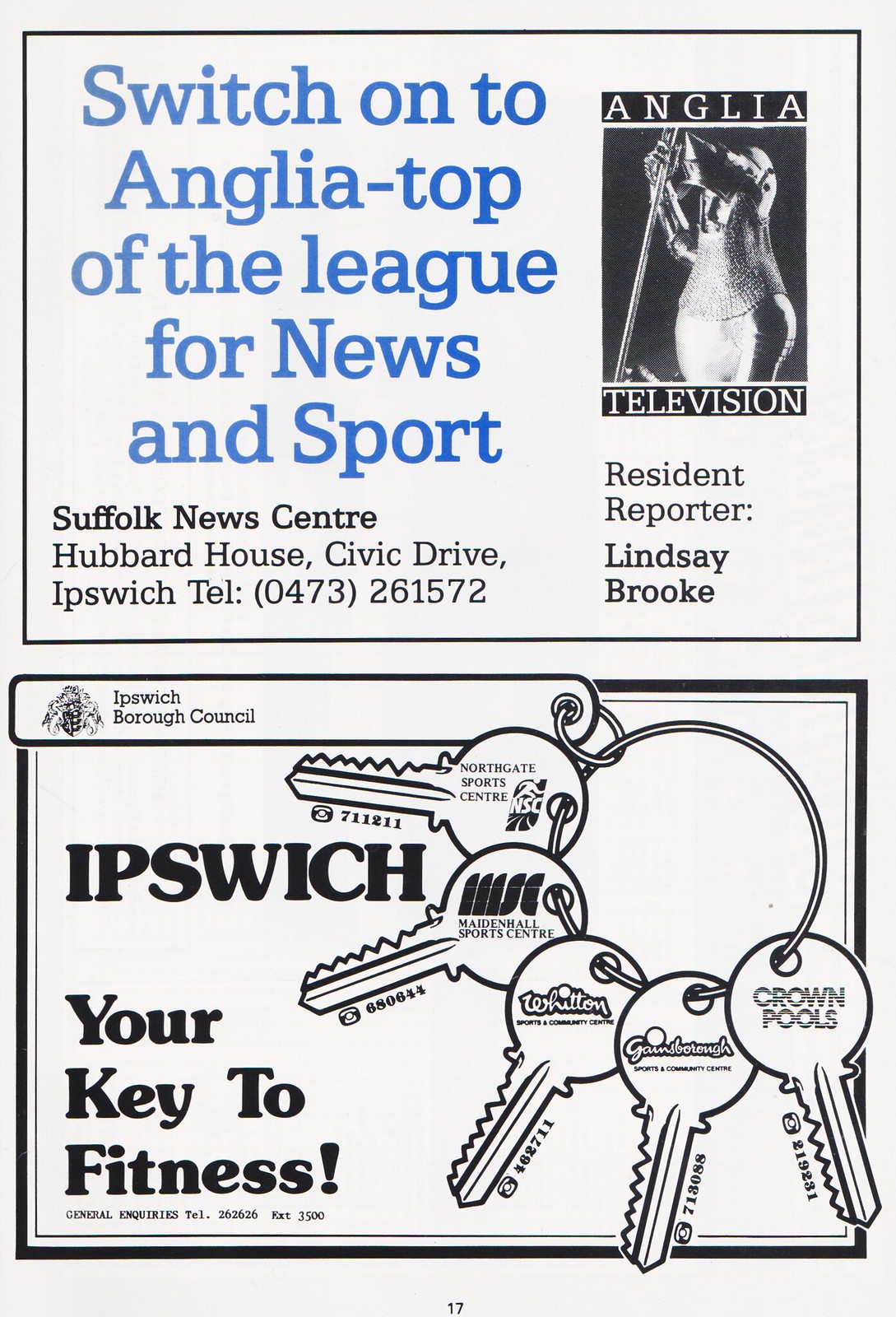The black and white business card prominently features detailed advertisements on both sides. The front of the card showcases a promotional campaign for Anglia Television, emphasizing its top-tier news and sports coverage. A striking image of a man clad in an old-timey chainmail battle suit serves as a visual centerpiece, complemented by the Anglia Television logo. At the top, in blue letters, it reads, "Switch to Anglia, Top of the League for News and Sports." This is followed by additional text introducing the resident reporter, Lindsay Brooke, and providing the address and telephone number for Suffolk News Center, Hubbard House, Civic Drive, Ipswich.

On the reverse side of the card, the focus shifts to an Ipswich Borough Council initiative. The design features a graphic of a key ring with five keys, each representing a different sponsor, including Crown Pools, Whitney, Garden Borough, and several sports centers. Dominating the bottom half of the card is the slogan "Ipswich: Your Key to Fitness," highlighting the community’s commitment to promoting health and wellness, bolstered by local business support.